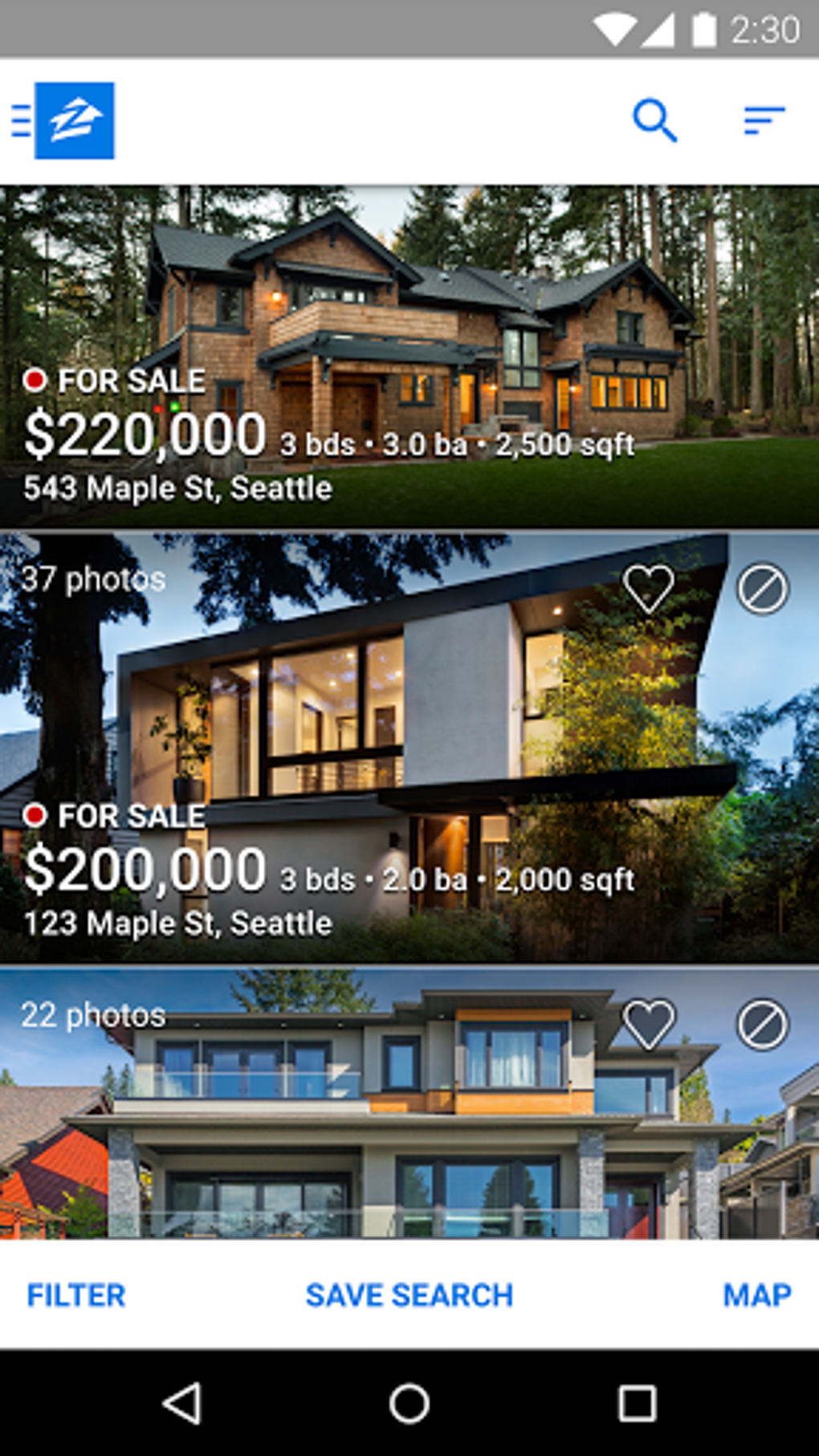This screenshot from a phone display depicts a real estate search interface, filled with multiple banners and detailed property listings. At the very top, a gray status bar shows generic phone indicators: a network symbol, a signal triangle, a battery icon, and the time "2:30". Just below, a white banner features an array of icons - three horizontal blue lines (likely a menu), a blue square, and a symbol of a "Z" within a white house.

Another white banner follows, containing a search icon and the same three blue lines. Below this, the main content shows three pictures of houses for sale:

1. The top image depicts a charming log cabin nestled in the woods, labeled as "For Sale: $220,000". Details listed include "3 BDS" (Bedrooms), "3.0 BA" (Bathrooms), "2500 SQFT" (Square Feet) at "543 Maple ST, Seattle".
   
2. The middle picture showcases a sleek, modern house. It features a beautifully sunny sky, and the property is characterized by its abundant glass windows and a flat roof, complemented by surrounding shrubs. The upper left corner mentions "37 photos". The listing reads "For Sale: $200,000" with "3 BDS", "2.0 BA", "2000 SQFT", located at "123 Maple ST, Seattle".

3. The bottom image presents another contemporary two-story house, dominated by glass windows and a second-floor balcony deck. The upper left corner indicates "22 photos". Below this image, there's a white banner with options: "filter", "save search", and "map" in blue.

The interface ends with a black banner, housing outlined shapes of a triangle, a circle, and a square.